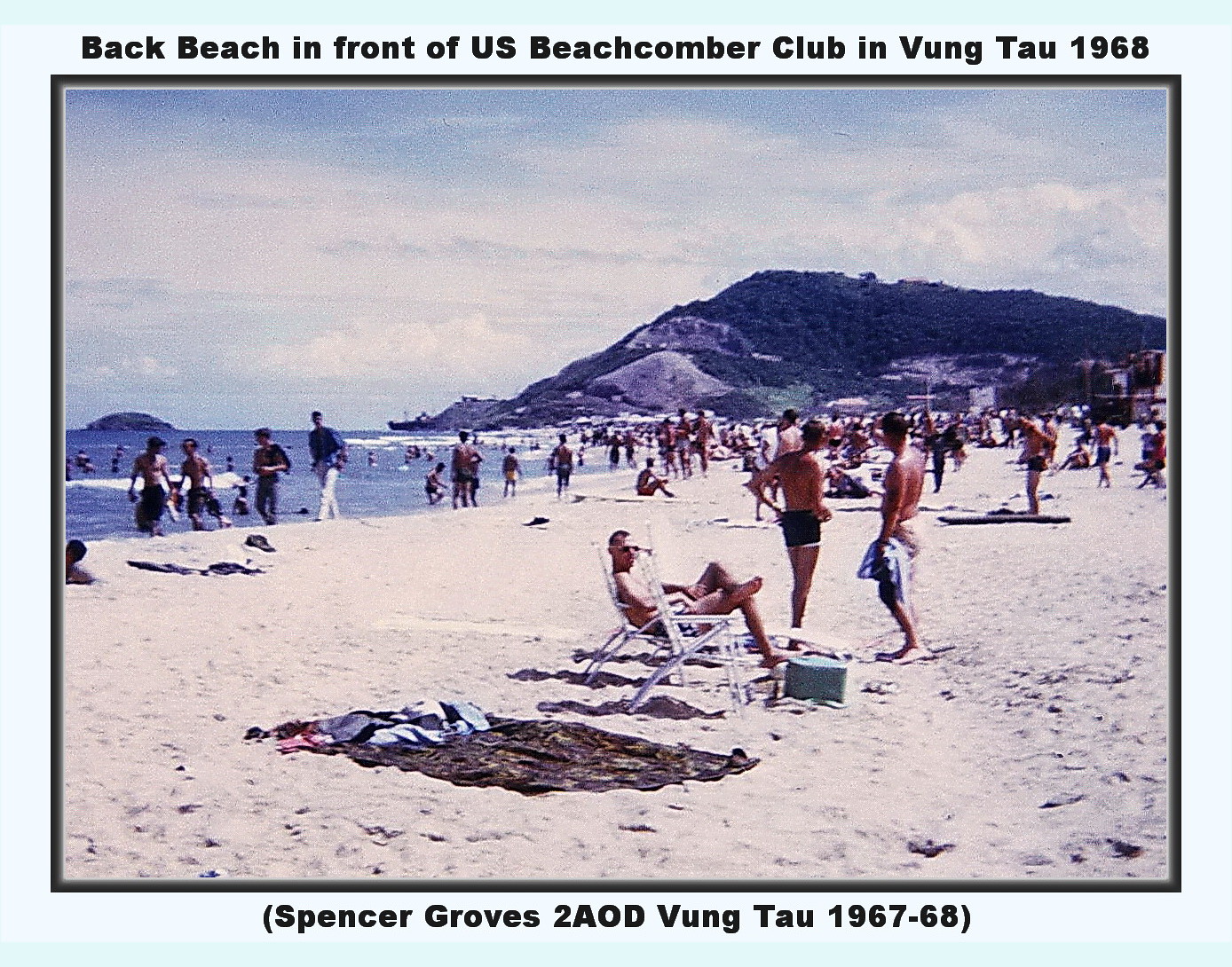The photograph depicts a bustling beach scene from 1968 in front of the U.S. Beachcomber Club in Vung Tau, as written in black text at the top. The muted and worn quality of the image indicates its age. The bottom of the image features the text "Spencer Groves 2-8 OD Vung Tau 1967-68" in black letters. White sands stretch across the beach, with a brown patterned beach towel prominent in the foreground. A man in swim shorts sits on a white lawn chair with a mint green box at his feet, flanked by two other men also dressed in swim trunks. The background reveals a lively crowd of 50 to 100 people, both clothed and in swimwear, with many standing, walking, or enjoying the water. A small green mountain rises from the coastline, enhancing the scenic backdrop.